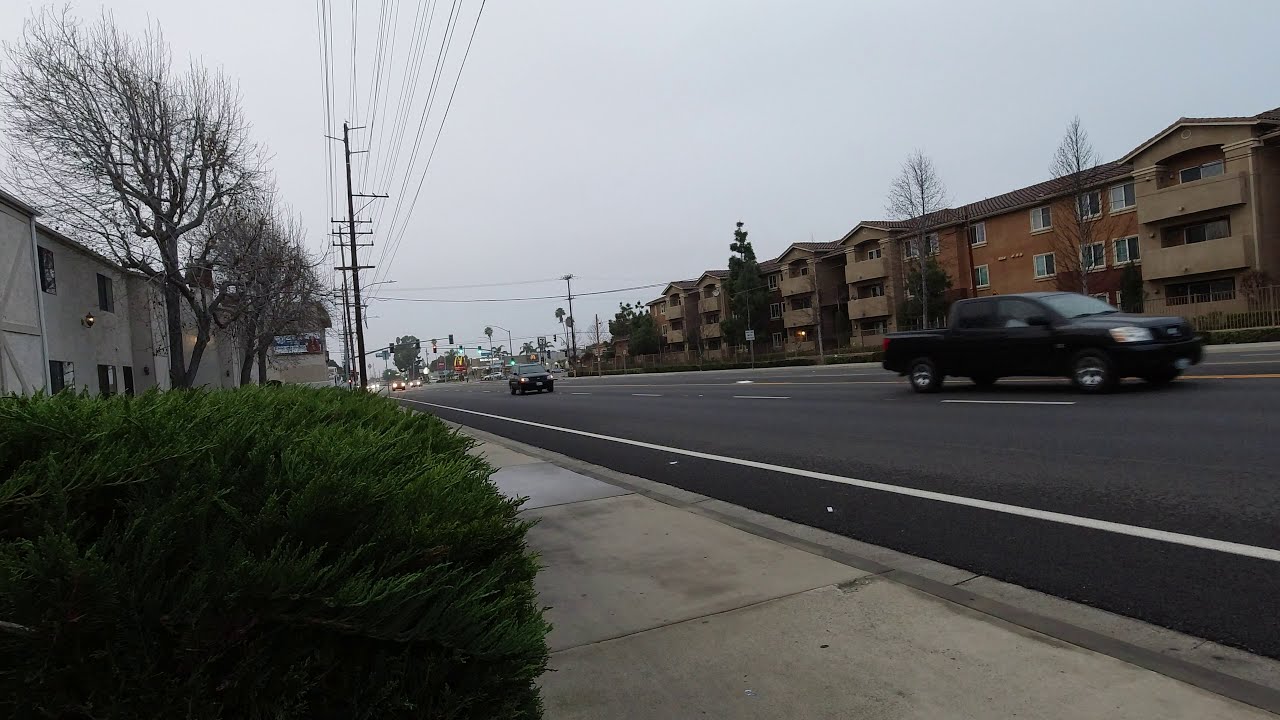This photograph, taken at street level on a cloudy evening, captures a segment of a small town street. Both sides of the four-lane road are flanked by apartment buildings with terracotta brick facades and balconies, while barren trees line the street. The road is marked with a central yellow dividing line and white lane stripes. The left foreground features a green evergreen shrub. A black truck is closest to the camera, followed by another black vehicle further down the road with its headlights on, emphasizing the twilight setting. In the background, a McDonald's sign and illuminated traffic lights indicate the presence of a busy commercial area, blending residential and commercial elements into this urban scene.